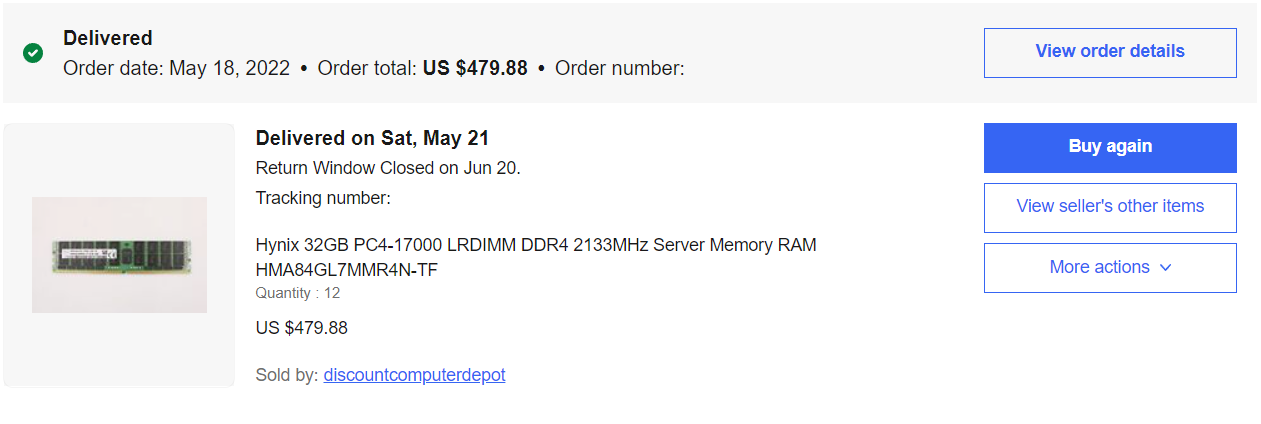This is a detailed screenshot of an order confirmation from an online retailer. At the top, a light gray background highlights the order status with a green circle and a white checkmark indicating "Delivered." Just below, the order date is listed as "May 18, 2022," and it is followed by a black dot separator. The order total is prominently displayed in bold as "US $479.88," separated by another black dot from the order number, which is not visible in the image. On the right side of this section, there is a blue-bordered box containing blue text that reads "View order details."

Beneath this header section, the background switches to white. On this white background is a gray square that houses a photograph depicting a single stick of RAM. The RAM stick is primarily green with black chips and a white sticker on the left side.

To the right of the photograph, there's detailed information about the order. The top line indicates the delivery status: "Delivered on Saturday, May 21." Accompanying this, it notes that the return window closed on "June 20," although there is no additional information attached to this note.

Below these details, the product information is listed: "Hynix 32GB PC4-17000 LR DIMM DDR4-2133MHz Server Memory RAM HMA84GL7MMR4N-TF." The quantity ordered is "12," and the total cost is reiterated as "US $479.88." The item is sold by "Discount Computer Depot," which is highlighted in blue and underlined, indicating a clickable link.

To the right of the product details, there are three action buttons. The top button is blue with white text that says "Buy Again." Below it, two blue-bordered buttons with blue text offer additional actions: "View seller's other items" and "More actions," with the latter featuring an arrow pointing downward, suggesting a dropdown menu.